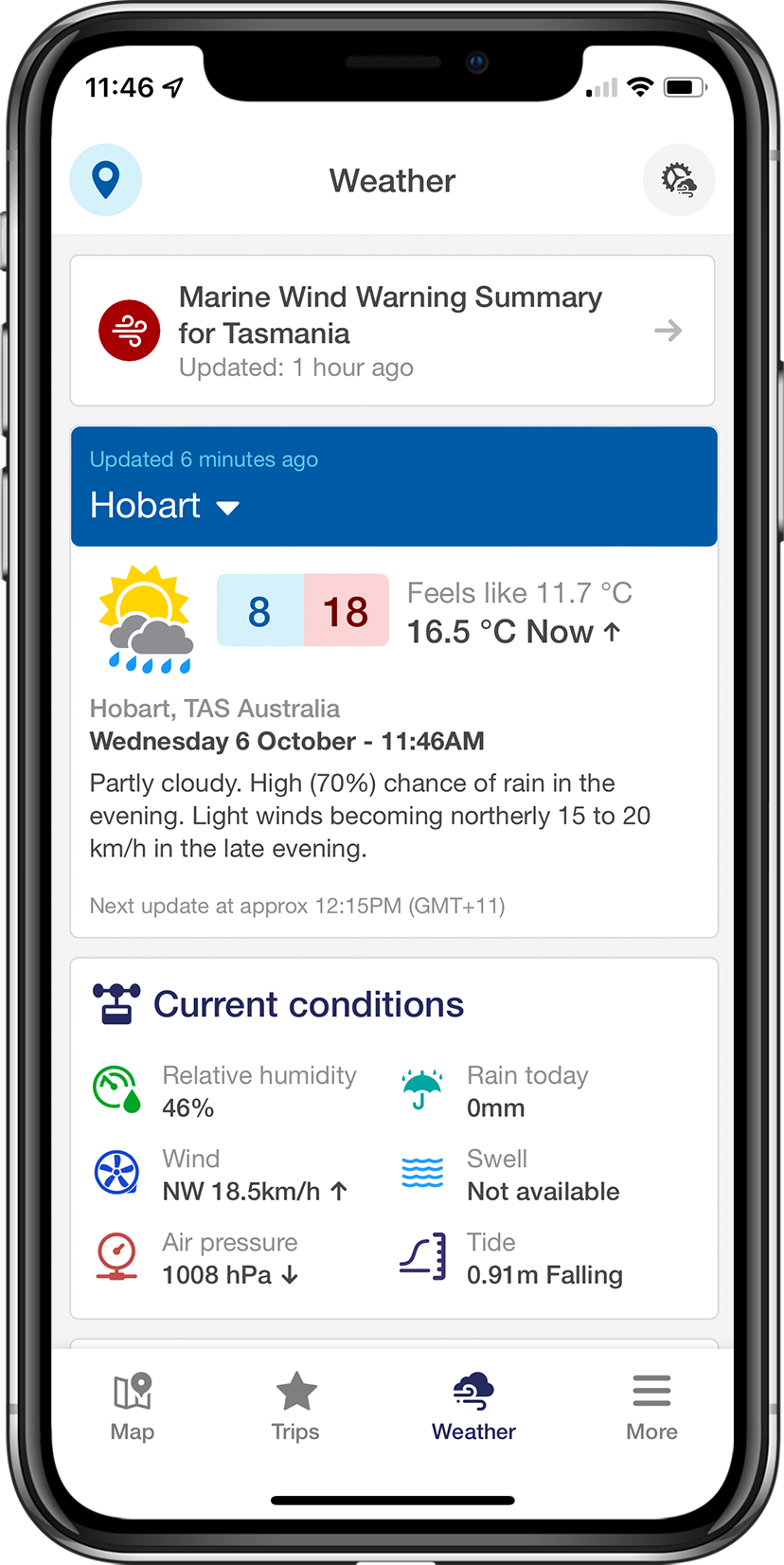This image is a mock-up of an iPhone displaying a weather app interface. The iPhone features include three buttons on the left side, a curved metal frame, and a front-facing camera situated in the top chin area. The status bar indicates the time as 11:46 AM, a single bar signal strength, and a battery level at approximately 75%.

The weather app interface showcases a variety of details:
- At the top, there is a weather icon with a location map pointer to the left and a gear icon to the right.
- A header below these icons, outlined in a thin gray pixel border, reads "Marine" and includes a small windy icon in a red, maroon circle. It alerts the user with a summary: "Maria Wind Warning Summary for Tasmania, updated one hour ago," accompanied by a right arrow.
- Beneath this, a blue field indicates an update from six minutes ago for Hobart, with a down arrow.
- The main weather condition graphic shows a sun partly obscured by two rainy clouds with water droplets. Adjacent fields, tinted in light blue and pink, provide additional data: "8:18 AM, feels like 11.7°C, currently 16.0°C, Hobart, TAS, Australia, Wednesday, 6th of October, 11:46 AM, partly cloudy with a 70% chance of rain, and light winds becoming northwesterly at 15 to 20 km/h in the evening."
- Current conditions detail 46% relative humidity, zero millimeters of rain, wind from the northwest at 18.5 km/h, unavailable swell information, air pressure of 1008 HPA, and a tide level of 0.91 meters and falling. Small corresponding icons are present next to each metric.
- At the bottom of the screen, navigation options include tabs labeled Map, Trips, Weather, and More.

The detailed layout provides comprehensive weather information for the specified location.